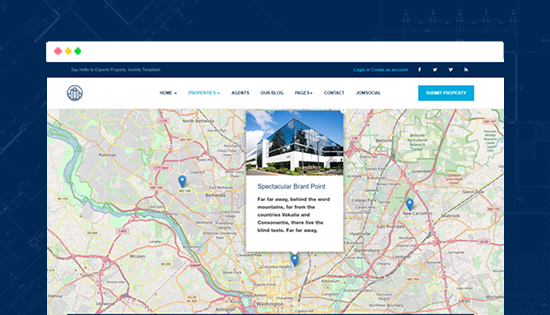This image showcases a webpage with a large map section prominently displayed, set against a navy blue background adorned with light gray lines crisscrossing it. Triangular shapes appear in the upper right corner of the background, adding a geometric touch.

The main webpage features a white bar at the top, decorated with small red, yellow, and green diamond shapes in the upper left corner. Beneath the white bar, various text, tabs, and buttons are present, including a login section and social media buttons on the right side.

Below these elements lies the main map. The map interface includes tabs such as "Home" and another tab that appears to be labeled "Contacts." There is also a notable blue button located in the upper right corner of the map section.

On the map, a specific building is marked, and a popup appears showing detailed information about this building, including a picture and additional details beneath it. This detailed layout provides easy navigation and information access through the website’s interface.